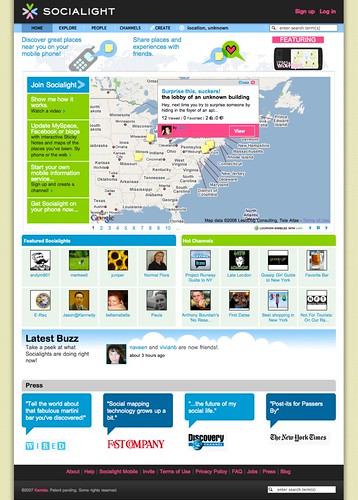A screenshot from the Socialite website prominently displays its user interface. At the top, a black bar spans the entire width of the screen, featuring the website name "SOCIALITE" in bold white capital letters on the left. Adjacent to this, a colorful logo composed of four hearts—colored blue, green, red, and yellow clockwise—forms a circle with their points facing inward. On the right-hand side, smaller red text options for "Sign Up" and "Log In" are visible.

Below the black bar, a blue navigation bar offers various clickable links, with the "Home" button highlighted in a darker blue, indicating it has been selected. Other links on this menu include "Explore," "People," "Channels," "Create," and another option that is not clearly visible. Toward the right, a white rectangle serves as a search box.

Occupying the main area beneath the navigation bar, the page predominantly features a large map depicting the eastern United States with labeled cities. To the map's left, a column of green boxes displays clickable links, each with white title text and black descriptive text. At the column's top, a blue box with white text invites users to "Join Socialite."

A central pop-up on the map shows a white-background box with black text reading "The lobby of an unknown building," followed by smaller descriptive text. A pink bar at the box's bottom contains a profile picture to the left and a "View" button in white on the right.

Beneath the map segment, two side-by-side sections present further content. The left section has a blue title bar with "Featured Socialites" in white text, and the right section features a light green title bar reading "Hot Channels." Both sections display two rows of four square profile pictures, each labeled with the channel name in blue text. The left section highlights individual people, while the right focuses on channels.

Further down, a thin section with a cartoon background of clouds and blue sky includes a "Latest Buzz" header in black text. Below it, smaller text invites users to "Take a peek at what socialites are doing right now." To the right, a square profile picture accompanies a notification showing that two people have become friends, identified in blue text with the remaining details in black text and timestamped "about three hours ago."

The final section features a grey title bar across the screenshot’s width, labeled "Press" in black on the left. Beneath this, four square speech bubbles alternate in light and dark blue, each with white text. The bubbles contain snippets of praise and commentary from various media outlets: "Tell the world about that fabulous martini bar you've discovered" from Wired (light blue logo), "Social mapping technology grows up a bit" from Fast Company (red logo), "The future of my social life" from the Discovery Channel (logo), and "Post-its for passers-by" from the New York Times (black text logo).

At the very bottom, a black menu bar offers links for help, contact, and terms of use, with red text and a final white rectangle search bar in the lower right corner.